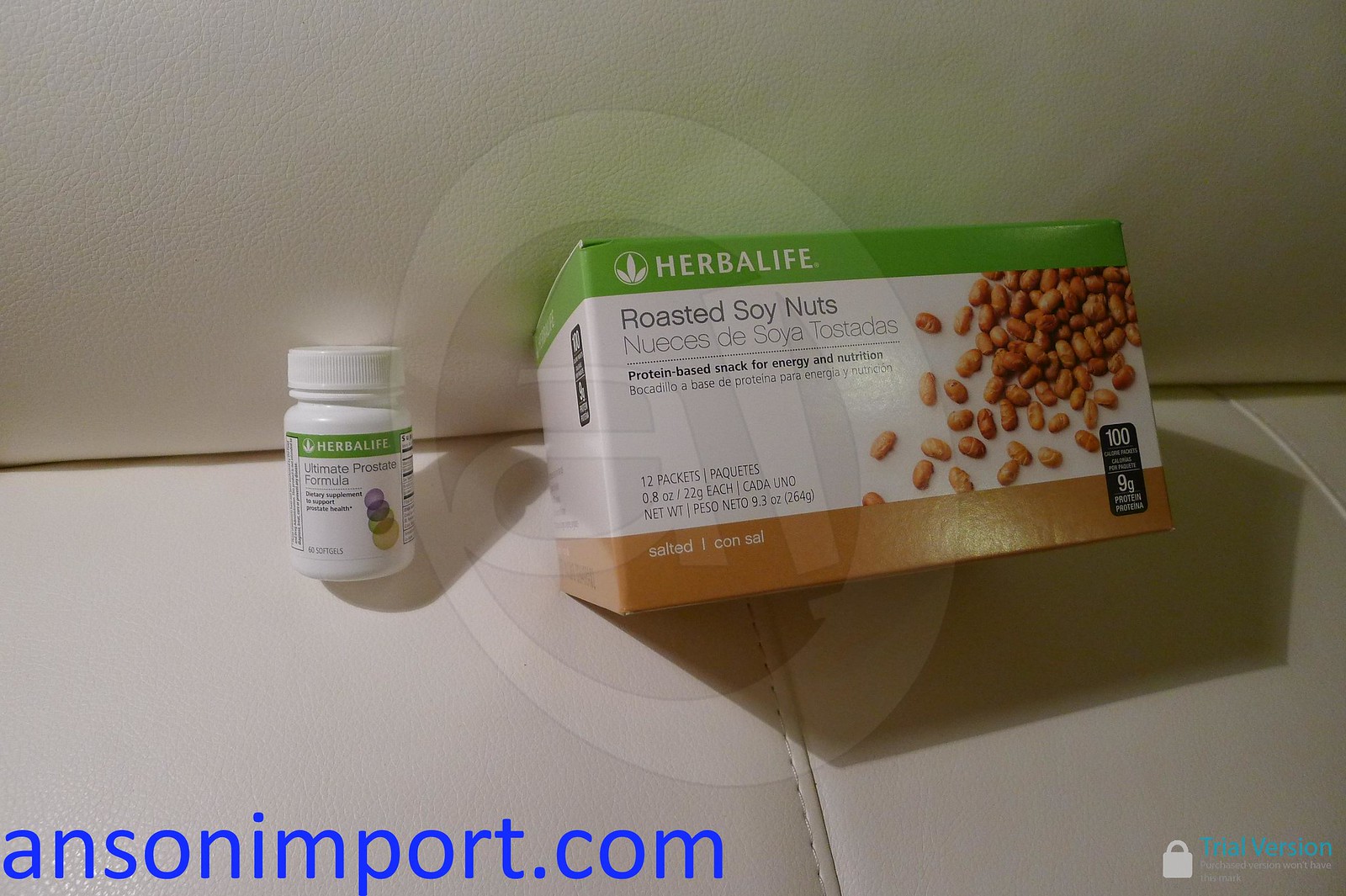The image depicts a product photo featuring Herbalife roasted soy nuts. Positioned on a white leather couch, the composition centers around two distinct packaging items. To the left, there is a small white bottle labeled with a green banner at the top reading "Herbalife." Below the banner, the label includes black text and an angled depiction of tablets presumably contained within the bottle. Adjacent to the bottle, on the right, stands a rectangular box with a green top displaying the "Herbalife" name and logo. The middle section of the box is white, prominently featuring the words "roasted soy nuts" alongside an angular image of the soy nuts themselves. The bottom section of the box, bordered in brown, specifies "salted" on the bottom left. The entire setting is framed by two watermarks: "AnsonImport.com" in large blue letters at the bottom center, and a "trial version" watermark positioned at the bottom right.